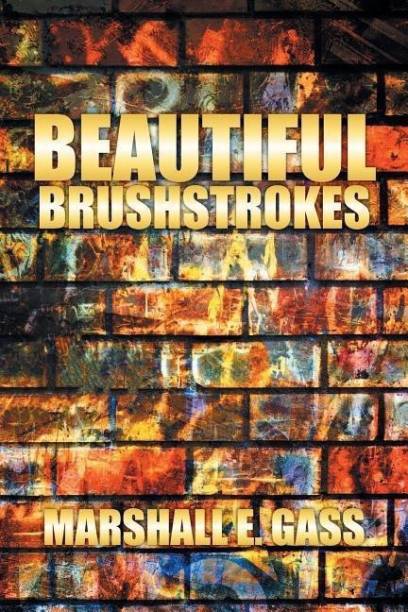This vibrant and artistic cover features a striking background composed of horizontally aligned bricks, each uniquely colored, creating a vivid and dynamic mosaic. The topmost rows transition from orange to brown, interspersed with white and blue bricks, leading down to a central blend of blue, white, yellow, gray, and brown. This colorful backdrop is layered with hues of black, red, green, purple, and additional streaks and shimmers, evoking a sense of movement and creativity. 

Prominently, at the top center of the cover, the word "BEAUTIFUL" is displayed in large, bold all-caps, accompanied by the word "BRUSHSTROKES" in a slightly smaller, but still bold, all-caps font, situated directly below. Both titles feature a light brownish-orange color with a striking horizontal yellow streak running through the middle, adding a mustard yellow gradient effect that transitions from darker edges to lighter centers.

Towards the bottom of the cover, the author's name, "MARSHALL E. GASS," is similarly styled in all-caps with the same yellow gradient and light brownish-orange coloration as the title text. The entire design gives off a graffiti-like impression, with vivid, brushed movements and gradient light effects across the brickwork, seamlessly blending into this eye-catching and art-inspired composition.